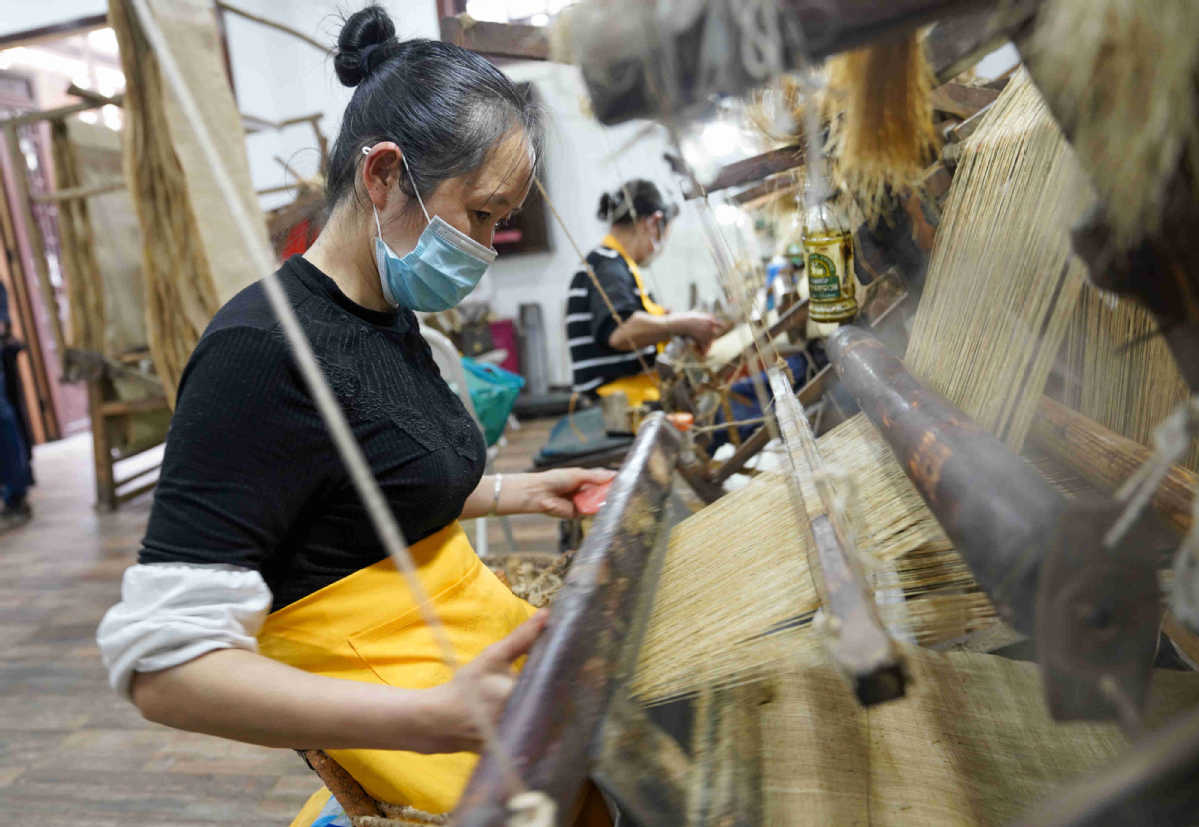In this photograph, two women are working on looms in what appears to be a bustling textile shop or factory setting, possibly during COVID times as they are both wearing masks. The woman in the foreground, who appears to be Asian, has her black hair tied up in a tight bun and is wearing a blue-and-white surgical mask that covers her nose and mouth. She is dressed in a black long-sleeve shirt with white accents, and over her clothing, she has a bright yellow apron. She is meticulously handling the intricate machinery of the loom, which is weaving beige threads, possibly crafting placemats. The environment looks crowded and somewhat cluttered, with a hardwood floor and various tools scattered around the large machines. In the background, another woman, also Asian with black hair in a bun, is similarly masked and attired in a black and white striped shirt under a yellow apron. She too is operating a loom, with the threads appearing to be of a similar beige color. Hanging fabric and a red door are visible in the background, suggesting a busy and productive space filled with textile materials.